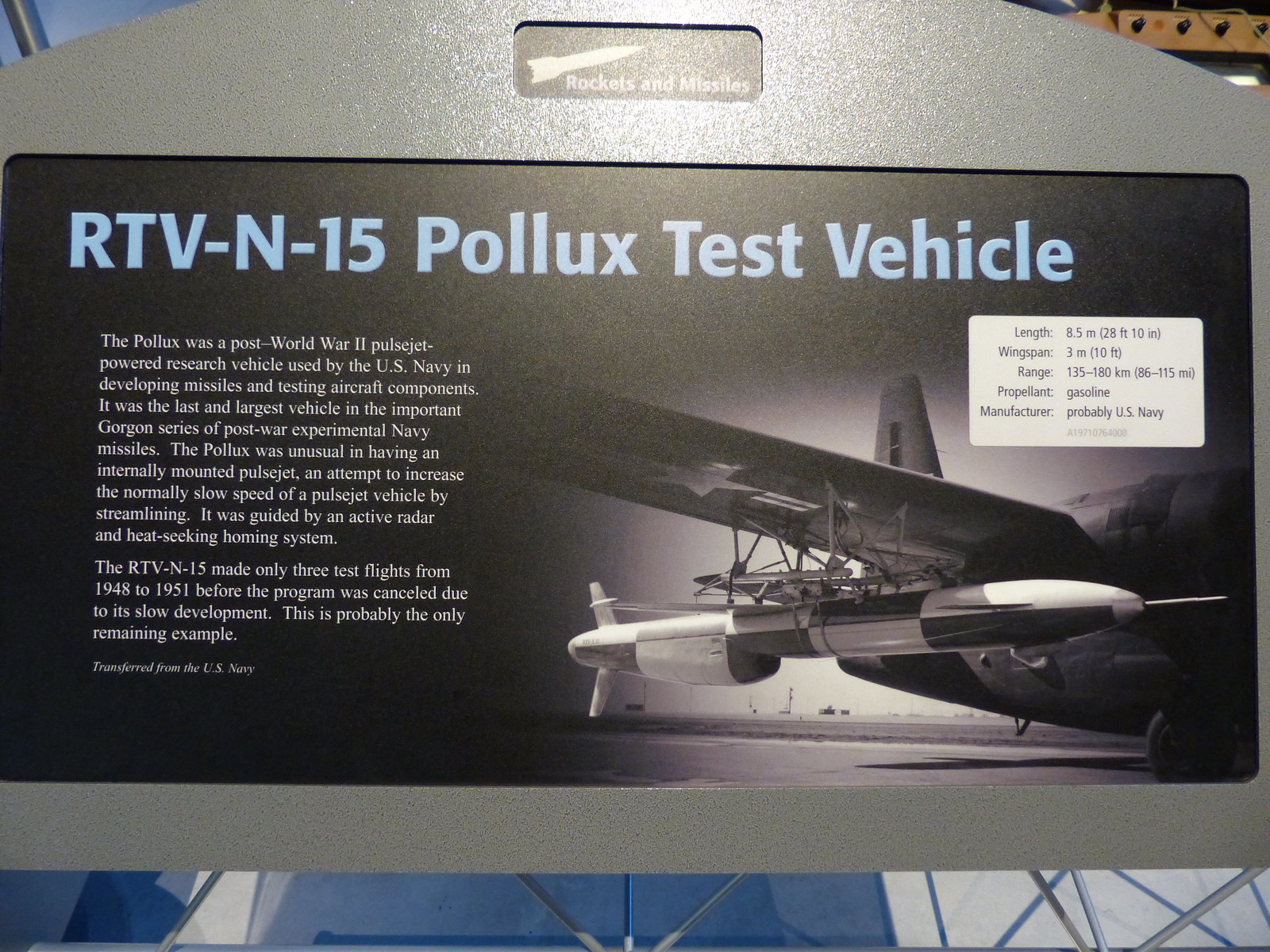The image captures a sign prominently displayed at what appears to be an air and space museum. The sign, which is centrally located in the photograph and possibly hanging amidst some visible scaffolding, provides detailed historical information about the RTV-N-15 Pollux test vehicle. The sign has a silver plastic frame with a large black rectangle in the middle. At the top of the sign, bold blue block text reads "RTV-N-15 Pollux Test Vehicle."

Beside the text, on the right-hand side, is a black-and-white photograph of an experimental aircraft, with a missile visibly mounted under its wing. Below the main heading in white font, a paragraph elaborates that the Pollux was a post-World War II pulse jet-powered research vehicle used by the U.S. Navy for developing missiles and testing aircraft components. It is noted for being the last and largest vehicle in the critical Gorgon series of post-war experimental Navy missiles. 

Further detailed information includes the dimensions of the vehicle, specifically mentioning an 8.5-meter length and a 3-meter wingspan, as well as a range of 135 to 180 kilometers. The paragraph explains the uniqueness of the Pollux, highlighting its internally mounted pulse jet aimed at streamlining to increase speed, guided by an active radar and heat-seeking honing system. It mentions that the Pollux underwent only three test flights between 1948 and 1951 before its cancellation.

The ornate black background on the sign contains several paragraphs of text that provide both technical data and historical context, emphasizing the vehicle's role and ultimate fate. This comprehensive exhibit appears to provide visitors with a deep understanding of the RTV-N-15 Pollux's significance in naval aviation history.